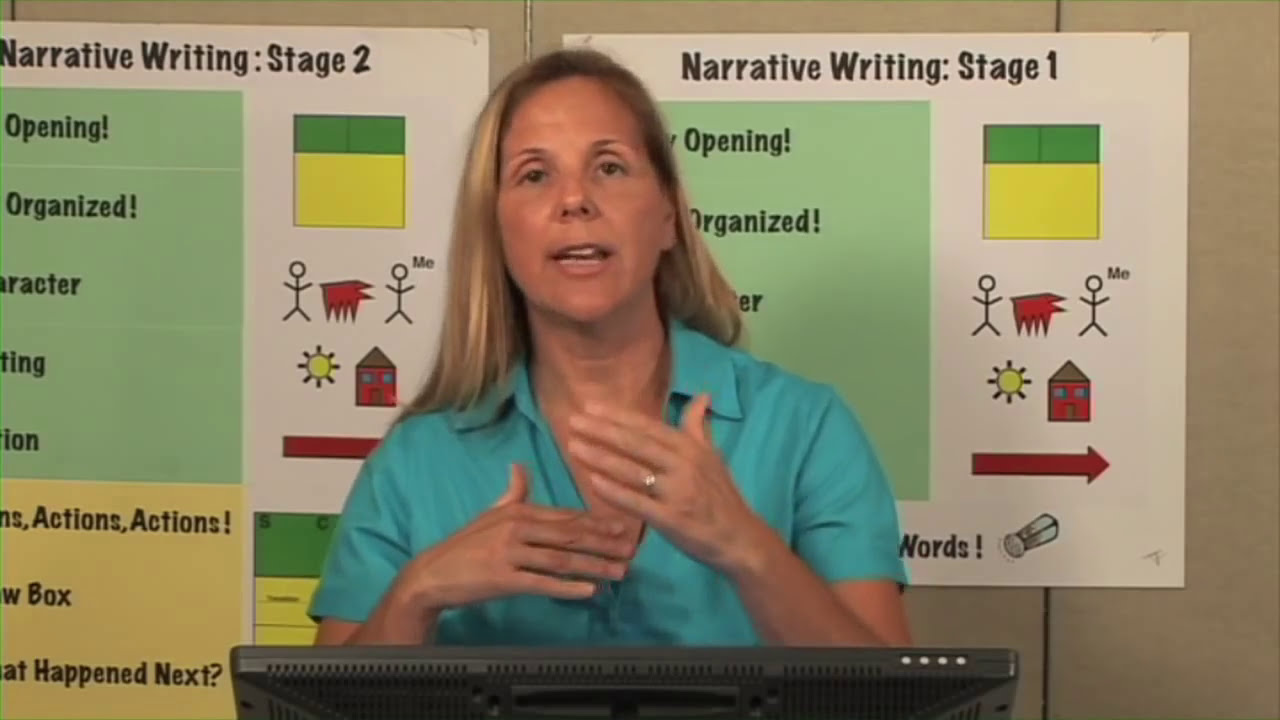In this screenshot likely taken from a video, a woman with long blonde hair and suntanned white skin stands centrally, actively engaging with the camera. She appears to be an educator, as her hands are raised in a demonstrative manner, mid-instruction. Behind her, two posters titled "Narrative Writing Stage 1" and "Narrative Writing Stage 2" suggest an educational context. The "Narrative Writing Stage 2" poster includes specific points such as "opening organized character" and "action," while the "Narrative Writing Stage 1" poster also starts with "opening organized." The woman, dressed in a short-sleeved teal blouse, stands in front of a monitor or screen, visible at the bottom edge of the image, likely containing the instructional materials she is discussing. The setting appears indoors against a tan-colored wall, reinforcing the impression of a classroom or lecture environment.